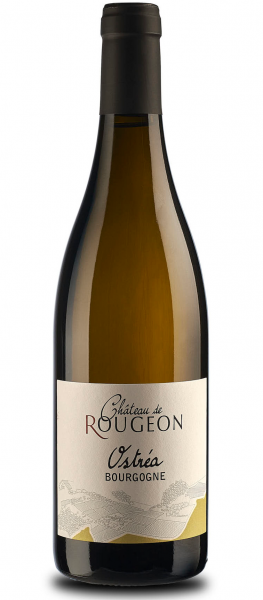The photograph features a beautifully presented bottle of Napa wine, specifically the Chateau de Rougeon. The bottle is placed against a plain white background, accentuating its elegant appearance. The wine bottle itself is tall with a thin neck that narrows towards the top and features a distinctive dark brown cork cap covered by a black ribbon. The glass of the bottle is a translucent dark hue, giving it a rich, burgundy tone. A prominent white square label adorns the front of the bottle, inscribed in fancy text with "Chateau de Rougeon" and "Austria Bourgogne" beneath it. The label's intricate design also includes artistic silhouettes of yellow and gray hills, hinting at a picturesque vineyard. The base of the bottle is the darkest part, further enhancing its robust appearance. The photo is a detailed, artistically edited representation, emphasizing the bottle's quality and sophistication.